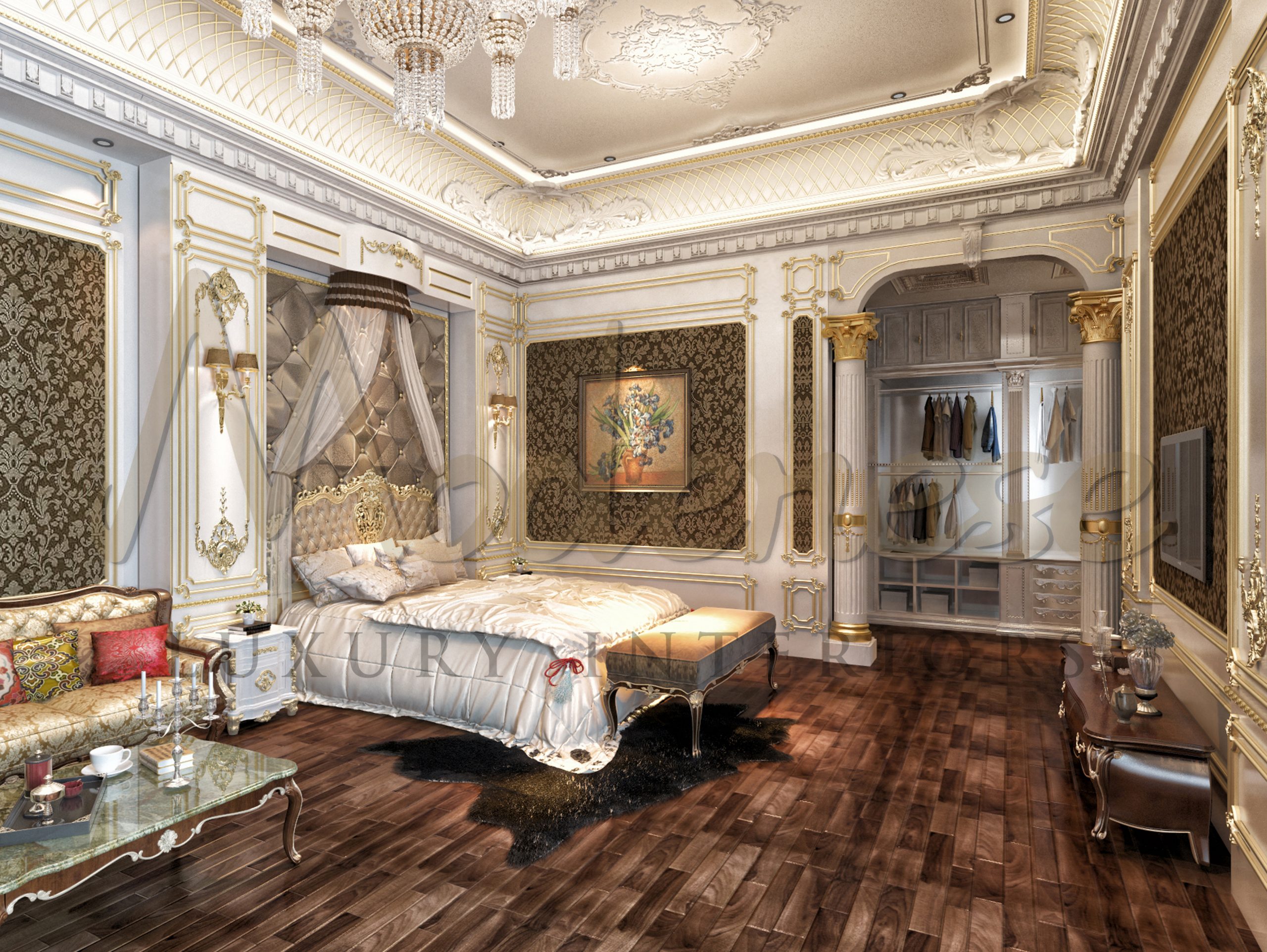This photograph showcases an opulent, vintage Victorian-style bedroom, characterized by a high tray ceiling adorned with an impressive crystal chandelier. The floor is a richly polished caramel walnut hardwood, amplifying the room's grandeur. On entering through white pillars with gold Corinthian tops, one notices the lavish decor, including extensive white and gold wood moldings and damask wallpaper featuring brown and gold hues.

The central piece is a queen or king-sized bed with a gilted silver-gold frame, adorned with a white satin duvet and pillows. Flanking this luxurious bed are silver curtains cascading down from a recessed wall. An ornate Louis XIV sofa in dark gold with white satin accents sits to the left, embellished with red and gold pillows. In front, a marble and wood coffee table holds a candelabra, teacup, saucer, and book.

The walls display intricate wainscoting with gold trim and rich wallpaper cutouts. Across from the bed, a short dresser rests below a mounted TV. A small bench sits at the bed's foot, enhancing the room's comfort. The open closet, visible beyond the pillars, contains neatly hanging clothes. Additional elements like a small table with a candelabra and a painting of flowers in a vase on one wall contribute to the room's luxurious atmosphere. A faint watermark reads "M-O-A-E-N-E-S-E luxury interiors," subtly overlaying this exquisite scene.